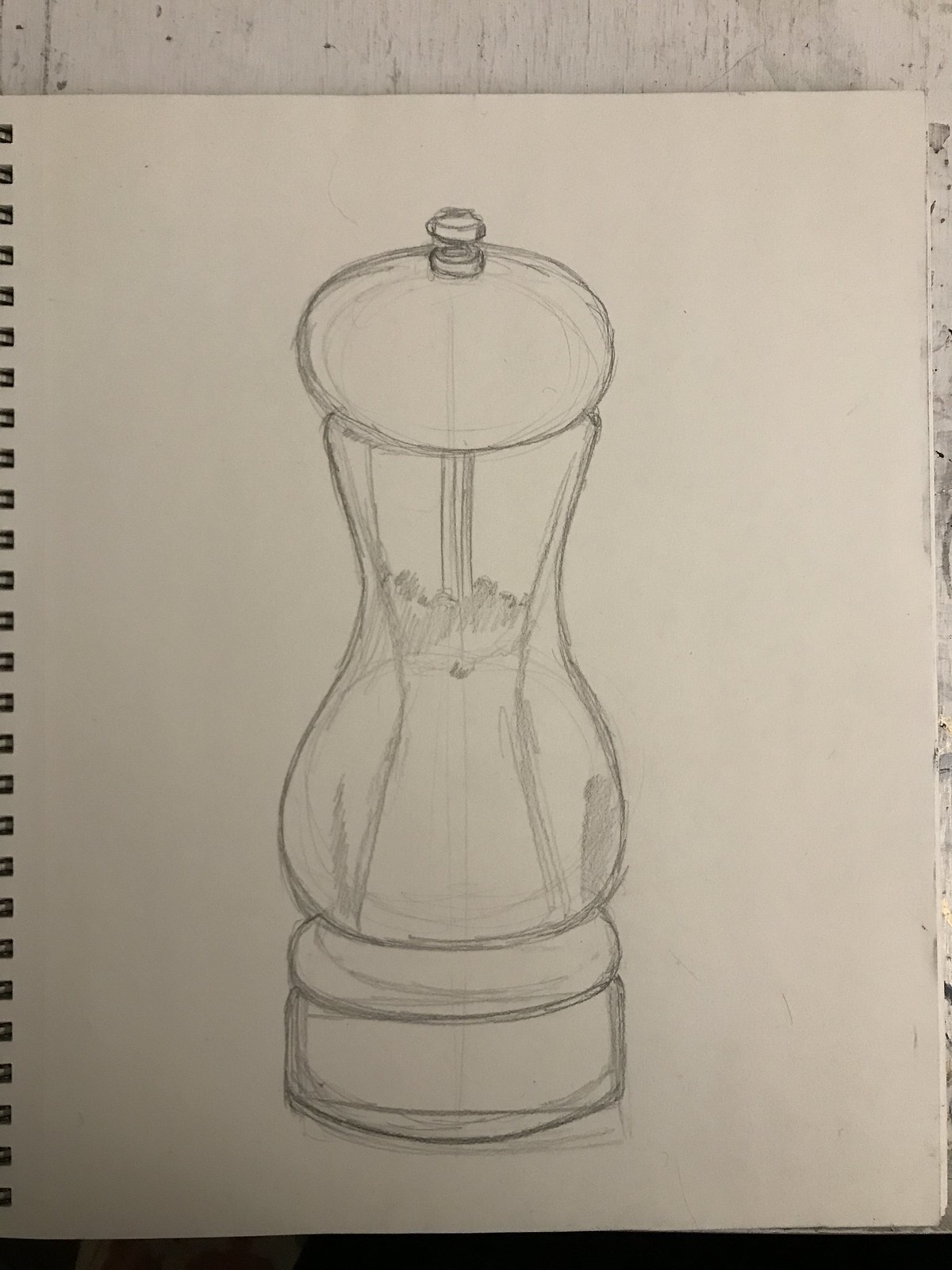This pencil sketch depicts a finely detailed pepper mill. The object features an hourglass-like shape, with a prominent, rounded top that resembles the classic knob found on traditional pepper mills. At the apex of this rounded top, there's a distinct circular bolt, typical of the functional design present in actual pepper mills. The middle section of the sketch subtly indicates small, round shapes, perhaps suggesting the internal grinding mechanism or peppercorns enclosed within. The base of the pepper mill is cylindrical, providing a stable foundation and completing the elegant, well-balanced form of the drawing.